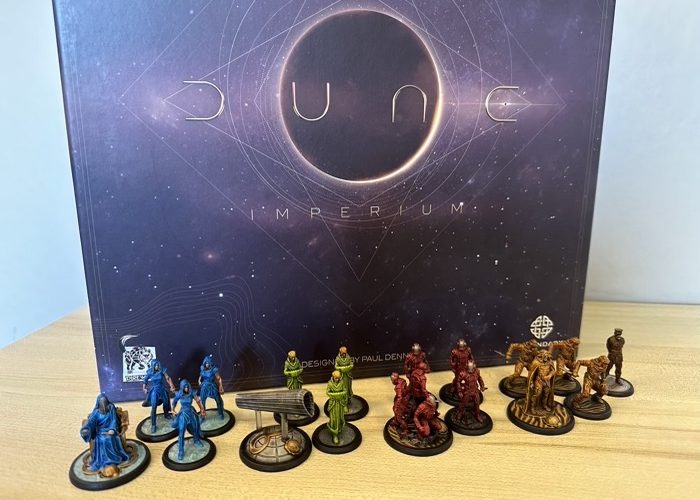This photograph showcases the board game "Dune: Imperium," with its box prominently displayed on a light wood table against a white wall. The box cover features the word "Dune" in silverish text, styled in the modern movie's typography, with 'Imperium' positioned below it. The background of the box art presents a cosmic night scene with black space and white stars. In front of the box are painted miniatures meticulously arranged: three blue figures to the left, three green monk-like figures nearby, and one green figure that resembles a floating log or cannon. There are four red figures grouped together, with an additional red figure towards the far right, and four yellow (or gold) figures. Finally, there is a single black figure positioned on the right. The detailed arrangement of these miniatures highlights the effort and skill in painting them, capturing the essence of the "Dune: Imperium" universe.